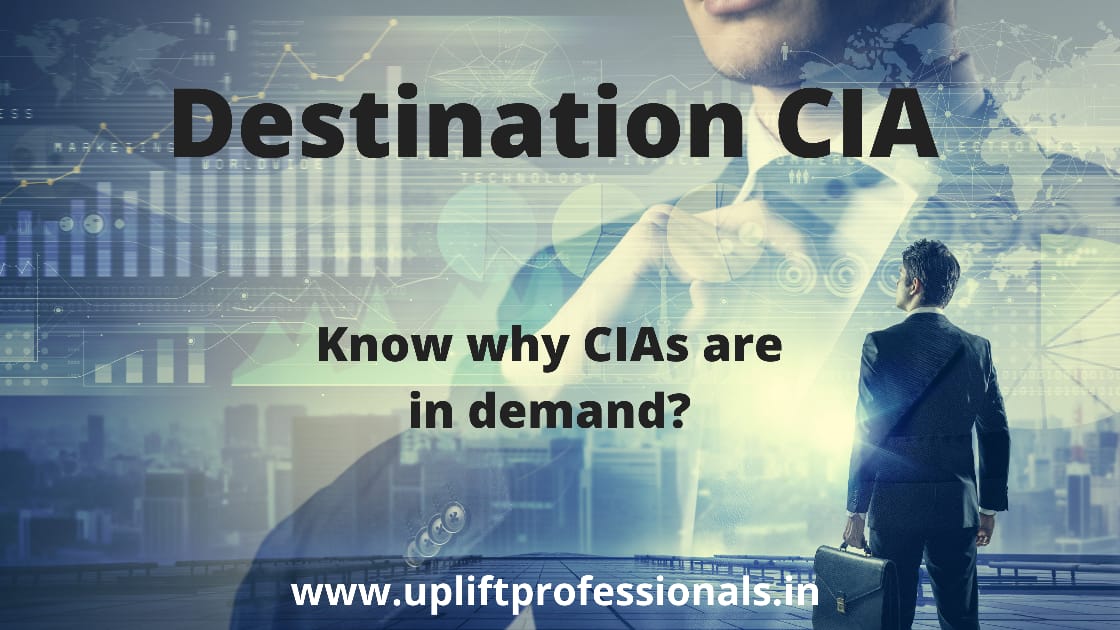The image features a detailed promotional graphic with a blue transparent background on the right side, showcasing a close-up of a man in a suit and tie, revealing his attire from below his bottom lip to his chest area. The left side of the image is filled with an array of data visualizations, including bar graphs, line graphs, pie charts, and a city skyline overlay. Additionally, various maps are visible in the background, enhancing the complex data-driven theme. 

Prominently displayed in large black lettering at the top center, the text reads "Destination CIA." Below this, still in large black text and centrally aligned, the image poses the question, "Know why CIA's are in demand?" 

At the bottom center, the website address "www.upliftprofessional.in" is written in white text. To the right of this text, the back of a man in a suit can be seen, holding a black briefcase in his left hand, suggesting a professional or corporate theme. The combination of these elements creates an intricate and somewhat enigmatic composition that seems to promote a professional service, despite raising questions about its legitimacy.